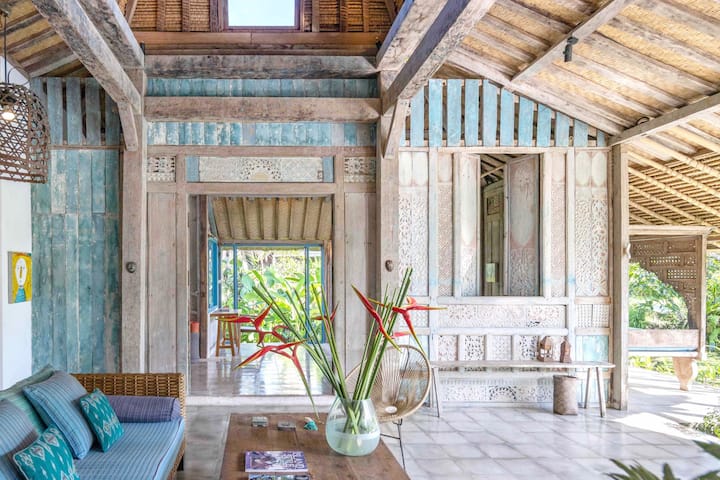The image showcases an inviting indoor-outdoor living space defined by its natural elements and seamless integration with nature. The interior of the house is designed with an abundance of natural sunlight streaming in through large, open areas where some walls appear absent. This open-space design is highlighted by the use of light beech wood across the walls, creating a warm, inviting atmosphere complemented by refreshing blue accents reminiscent of water. Central to the room is a round table featuring a massive plant in a glass vase, emphasizing the natural theme.

In addition to the main living area, the scene extends to an outdoor patio that mimics a cozy living room. This patio area features a blue couch adorned with pillows, positioned near a table that holds several magazines. The floor is laid with natural tile, and the patio itself is primarily constructed of wood, including both brown and white wood elements. The presence of various plants and trees both within and surrounding the patio area enhances the connection to nature, further supported by the greenery visible in the background. Mirrors and other decorative elements add to the aesthetic appeal of this serene, nature-oriented living space.